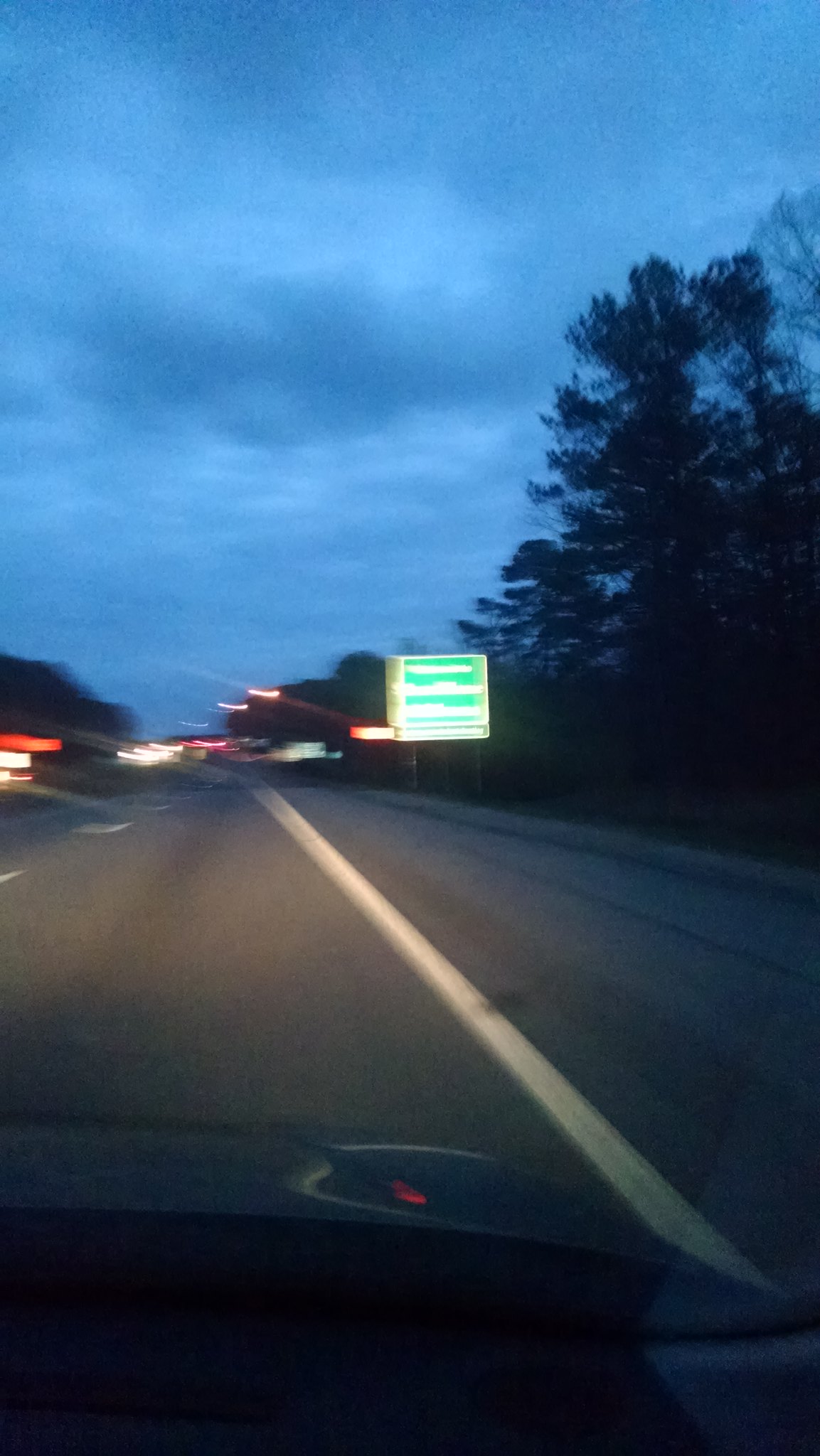The image is a blurry photograph taken from the passenger seat of a car, likely captured by a dash cam. The scene depicts a multi-lane highway, distinguished by white lines marking the spacious lanes and a white shoulder separated by a distinct stripe. The roadside features a green sign with white lettering on the right-hand side, but the text is unreadable due to the blurriness. The time of day appears to be either early morning or late evening, given the darkening sky with hues of blue and white. The highway is dimly lit, with the presence of trees along the roadside, and a few illuminated buildings are faintly visible in the background. This setting, combined with the sky transitioning to nightfall, gives the scene an overall dim and indistinct appearance.